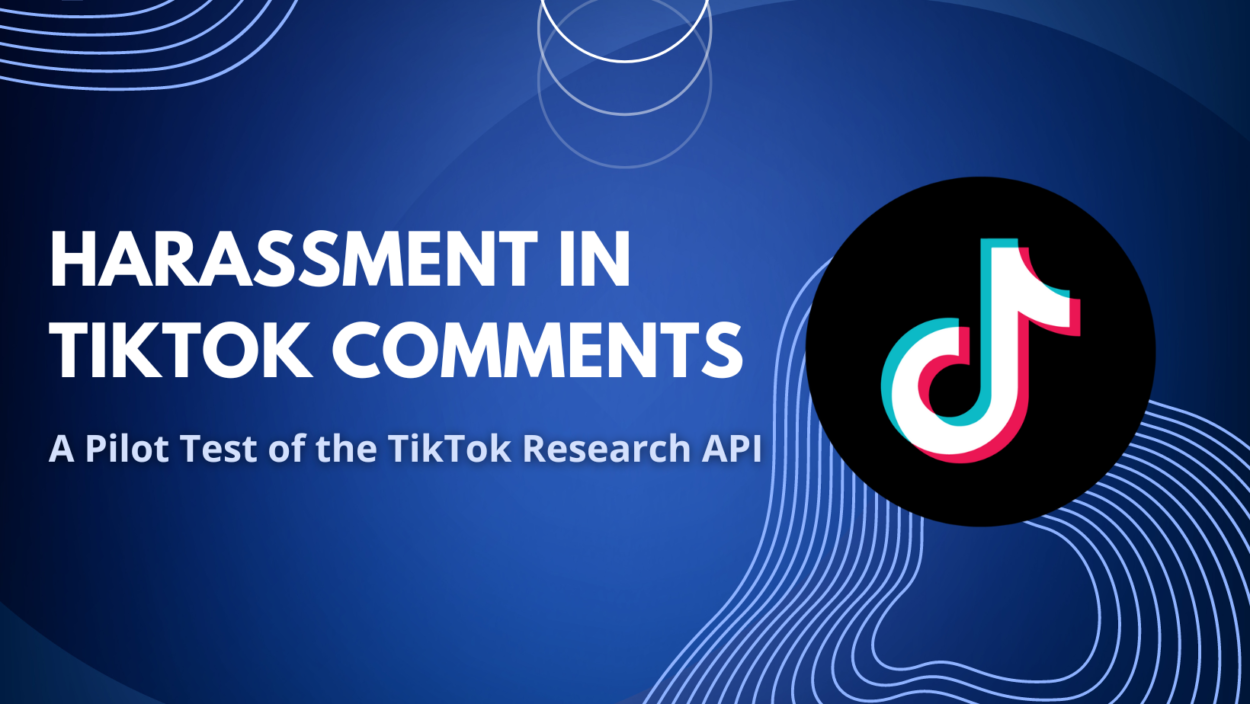The image features a dark blue rectangular background, adorned with white, curvy lines reminiscent of topographical map features indicating distance and elevation. These lines are concentrated in the top left and bottom right corners, creating layered, round shapes. In the top middle part of the image, there is a cluster of three concentric circles. Additionally, the top right and lower left sections of the image are shaded in a lighter blue hue, contrasting with the predominant dark blue.

Central to the design, in bold white capital letters, is the word "HARASSMENT," followed by "TIKTOK CONTENT COMMENTS." Below this, in smaller, grayish lowercase letters, it reads "A pilot test of the TikTok Research API." Positioned to the right of the textual content is the TikTok logo, a distinctive black circle featuring a multicolored symbol resembling a musical note or an upside-down letter "P," in shades of blue, purple, white, and pink.